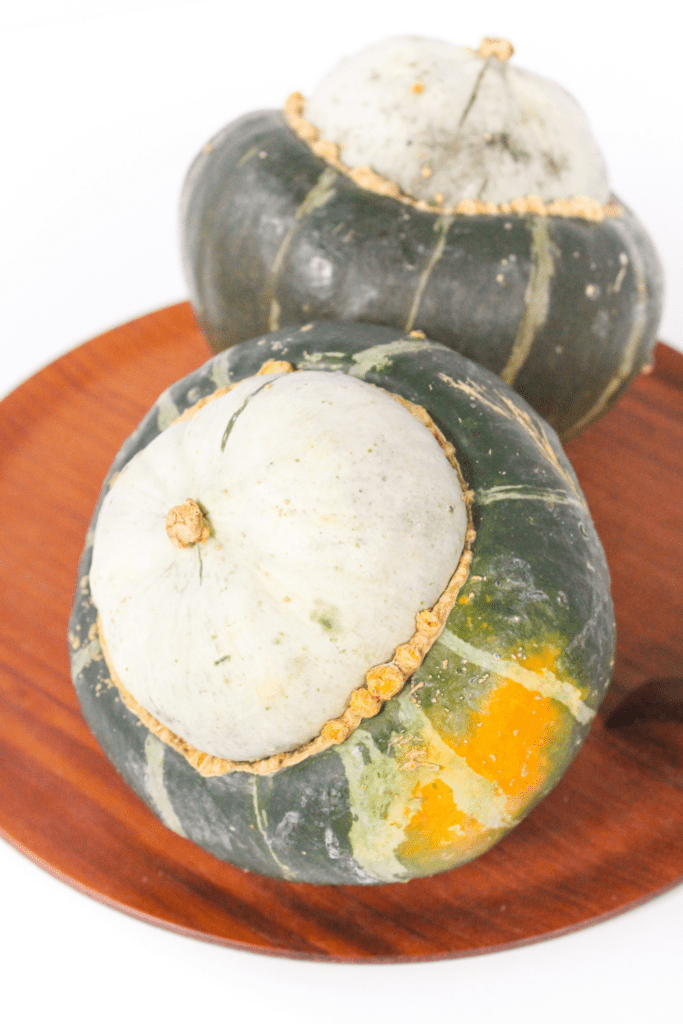The image features two acorn squashes resting on a circular wooden board with a light, medium brown grain. The edges of the board are truncated, leaving the top hidden by the vegetables and the sides cut off. Both squashes are primarily dark green with light green or whitish vertical stripes. The tops of the squashes have a very light green to white "cap" area, where stems were previously attached, one showing a splotch of yellow or pale orange where sunlight didn't reach during growth. The squash in the front leans to the left with an orange spot on its lower right side, partially overlapping the one behind. The rear squash, smeared with some dark dirt on its cap, tilts slightly back and to the right. The background, apart from the wooden board, is white, accentuating the vivid colors and textures of the squashes.